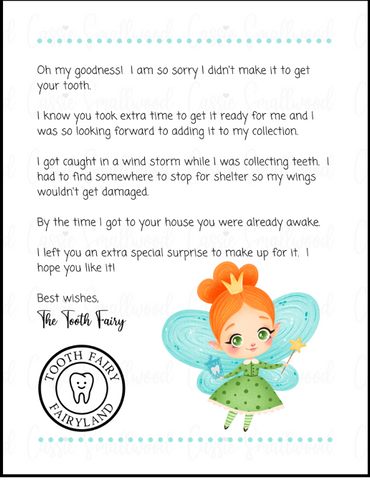The flyer features a detailed apology note from the Tooth Fairy, set against a white background with a thin black border and dotted blue lines at the top and bottom. The text reads:

"Oh my goodness, I am so sorry I didn't make it to get your tooth. I know you took extra time to get it ready for me and I was looking forward to adding it to my collection. I got caught in a windstorm while I was collecting teeth. I had to find somewhere to stop for shelter so my wings wouldn't get damaged. By the time I got to your house, you were already awake. I left you an extra special surprise to make up for it. I hope you like it. Best wishes, The Tooth Fairy."

In the bottom right corner, there is a charming illustration of the Tooth Fairy. She has orange hair styled in a bun, adorned with a gold crown. She wears a green dress with darker green dots, paired with green and white stockings. Her fairy wings are large and blue, and she holds a brown wand topped with a yellow star. To the left of the fairy, there is a stamp-like circle featuring the text "Tooth Fairy, Fairyland" and a cartoon tooth at its center.